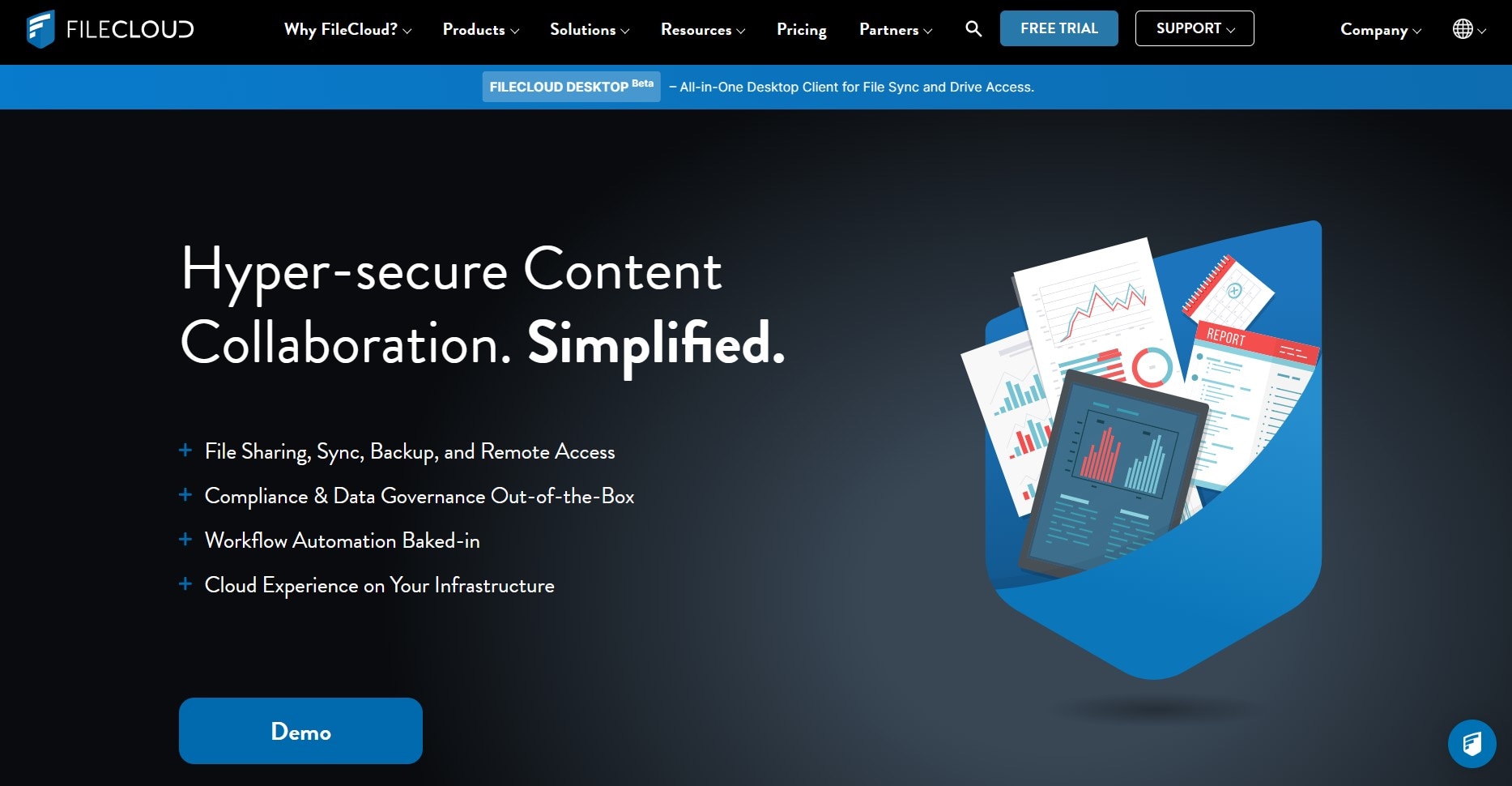The website homepage for FileCloud features a comprehensive and well-organized layout designed for ease of navigation and accessibility of key information. At the top of the page, the header prominently displays "Why Choose FileCloud" with a dropdown menu for additional details. The header includes sections such as Products, Solutions, Resources, Pricing, and Partners, each providing further insights through dropdown menus.

The FileCloud logo is situated within a black horizontal bar that extends across the page, and features reverse print in white. To the left of the logo is a small badge-like icon with white horizontal lines.

Adjacent to the Partners section, users will find a search icon represented by a magnifying glass, allowing for easy content discovery. Further to the right, a blue button offers access to a free trial for those not ready to commit financially. Additional options include Support and Company, each with their own dropdown menus, and an option to change the language of the website.

Beneath the header is a banner introducing the FileCloud Desktop, currently in its beta version. It is promoted as an all-in-one desktop client for sync and drive access. An accompanying image shows various charts emerging from a pocket, visually suggesting the tool's analytical capabilities.

To the left of this image, bold white text declares "Hyper Secure Content Collaboration Simplified." Below this statement, a series of bullet points with plus symbols highlights the key features: File Sharing and Sync Backup, Compliance and Data Governance, Workflow Automation, and an Integrated Cloud Experience.

A prominent demo button is located just beneath these feature descriptions. At the bottom right corner of the page, a small icon resembling a chat bubble suggests the availability of live support, though it is not explicitly labeled.

Overall, the website is designed to be user-friendly and informative, providing prospective users with immediate access to vital features and support options.